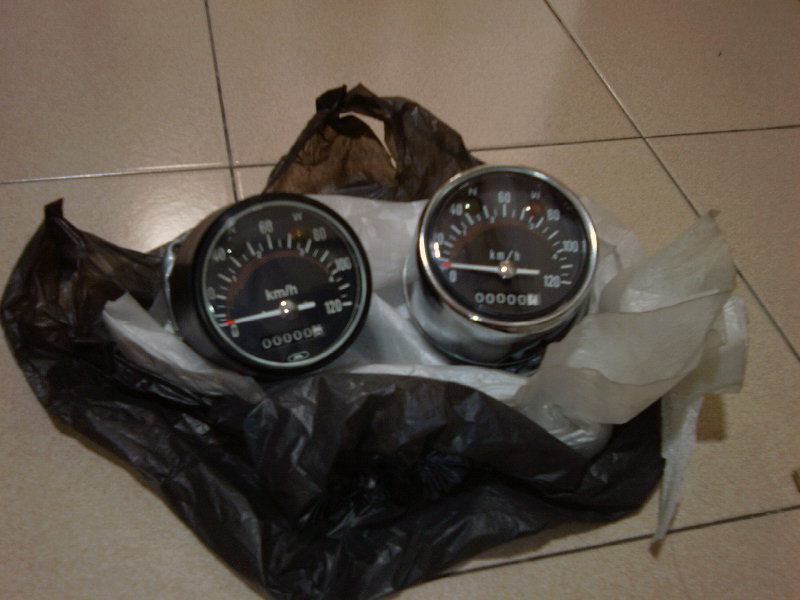The image features two speedometers placed atop a white plastic bag, which is itself resting on a round grocery plastic bag. 

The speedometer on the right is encased in a silver, relatively thick bezel and displays zero miles on the odometer. It features a white needle and two small, indistinct dots on the glass cover. The face of the speedometer is black with white markings, indicating measurements in kilometers per hour. The number seven is visible next to the "000000" mileage indicator.

In contrast, the speedometer on the left is shorter in stature and has a black casing. This too shows zero miles on the odometer, with a black face and white lettering. Both speedometers have white markings for speeds in kilometers per hour.

Beneath the speedometers, the white plastic bag has dirty, ripped edges. The entire setup is on a large, cream-colored tile floor with visible gray grout lines.